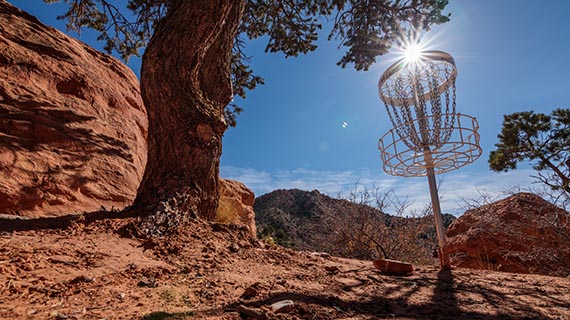This photograph captures a sunlit, rocky desert landscape, characterized by dark brown and red clay soil that permeates the ground. Prominently in the scene is a silver frisbee golf goal, comprising a metal pole with a circular basket near the middle, and chains hanging from a circular ring above, designed to catch discs. This pole appears to lean slightly. To the left stands a large, curved tree with a distinctive hole in its trunk, its branches adorned with green leaves. Nearby, a tall, dark brown rock adds to the rugged terrain. In the background, two smaller hills of red clay are visible, with one showing a protruding tree limb and the other dotted with additional greenery. The sky above is a clear blue with minimal clouds, and the whole scene is bathed in bright sunlight, casting shadows of the trees and the frisbee golf goal on the ground.